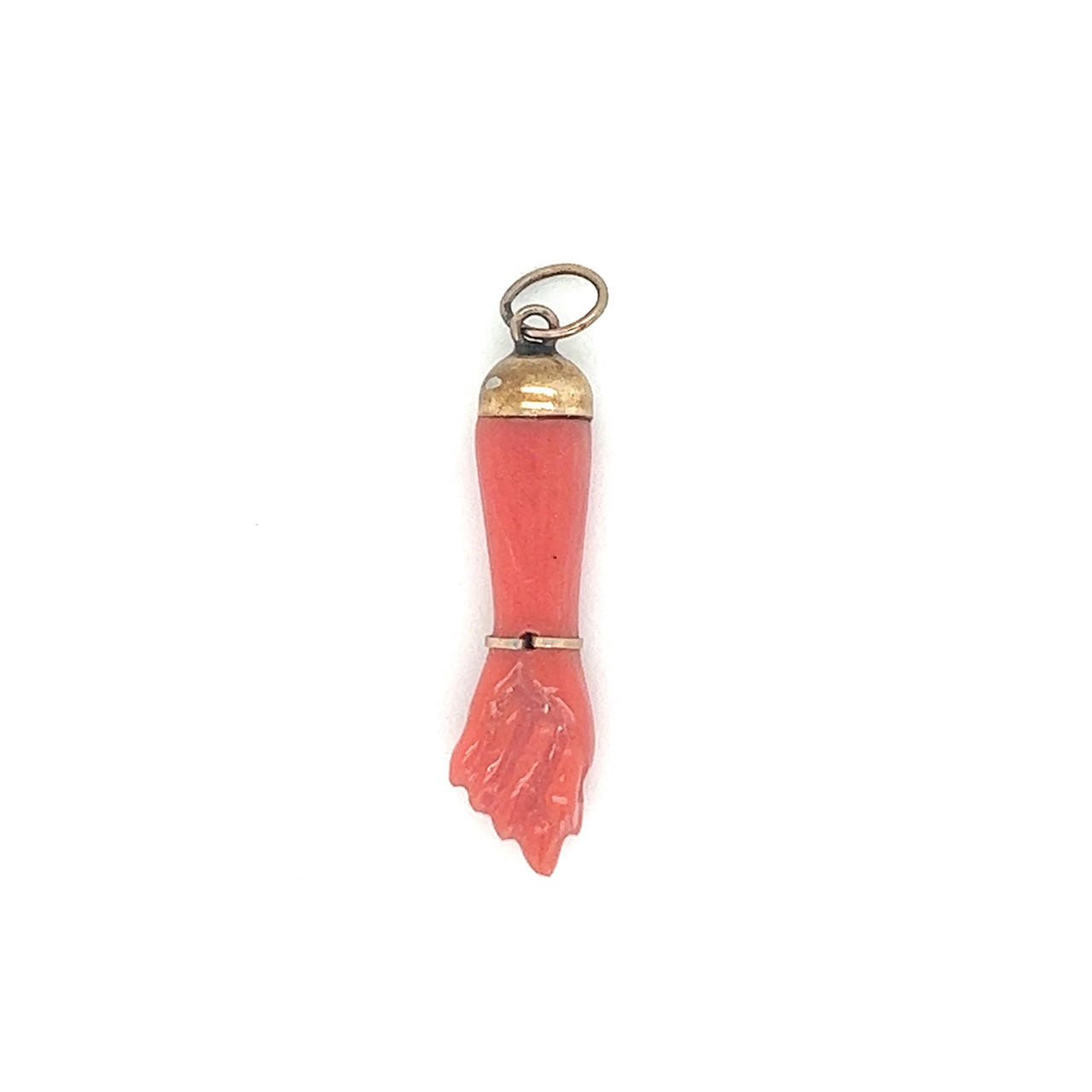The image features a polished charm resembling a human hand balled into a fist, made from a stone-like material colored pale pink, somewhat akin to a melted Jolly Rancher candy. The charm is intricately detailed, with discernible, though not separated, fingers. The fist points downward, held within a golden, slender, rectangular bracelet-like band encircling the wrist area, adorned with a small dark square. Above this band, a silver cup forms the top end of the arm, from which emanates a circular golden loop for attachment. The background of the image is solid white, enhancing the charm's unique colors and details. The arrangement suggests the charm could function as a keychain or an ornamental accessory.